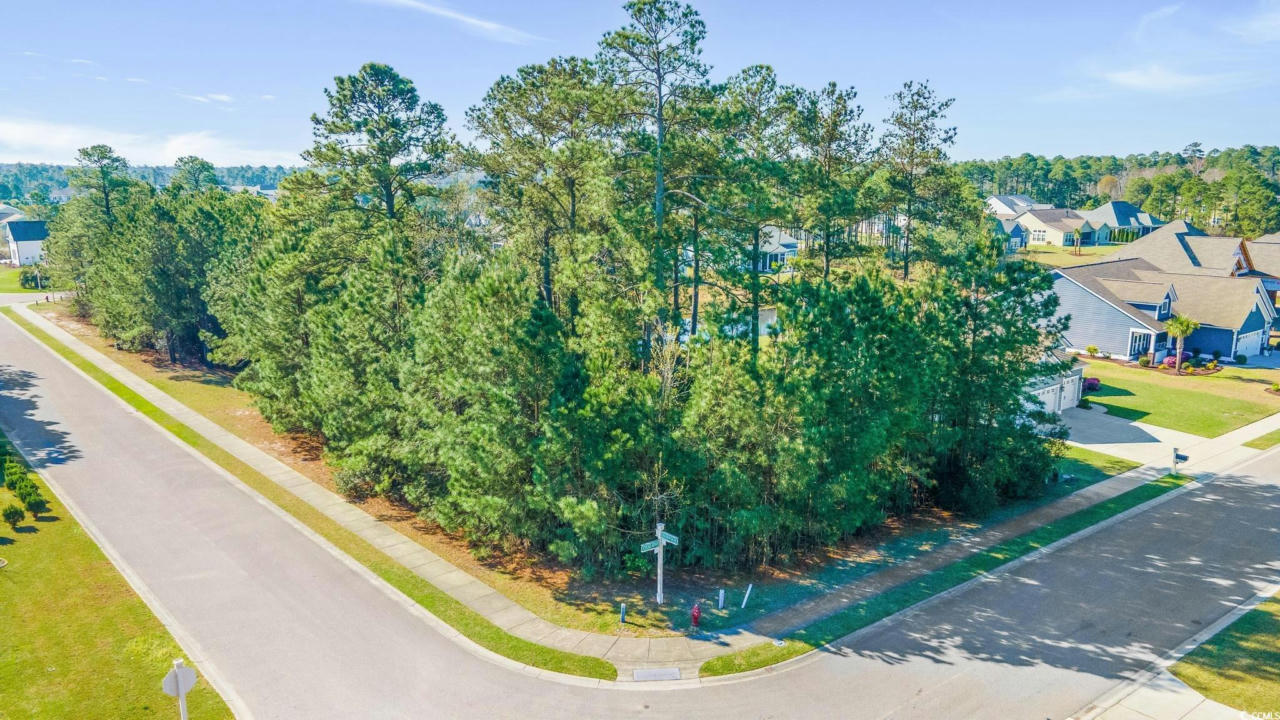The image depicts a street corner in a suburban neighborhood, viewed from a high perspective. The intersection features two roads forming a V-shape, with a sidewalk running along the upper side and curving toward the right. A red fire hydrant is positioned near the corner, in front of an area with green shrubbery and tall trees. A street sign is also present at the intersection, though the street names are not legible. The background shows houses with well-kept green lawns, primarily blue with brown roofs or white in color, some with driveways intersecting the sidewalk and leading to garages. The scene is bathed in light under a blue sky with a few wispy clouds, capturing a peaceful and well-maintained suburban setting.